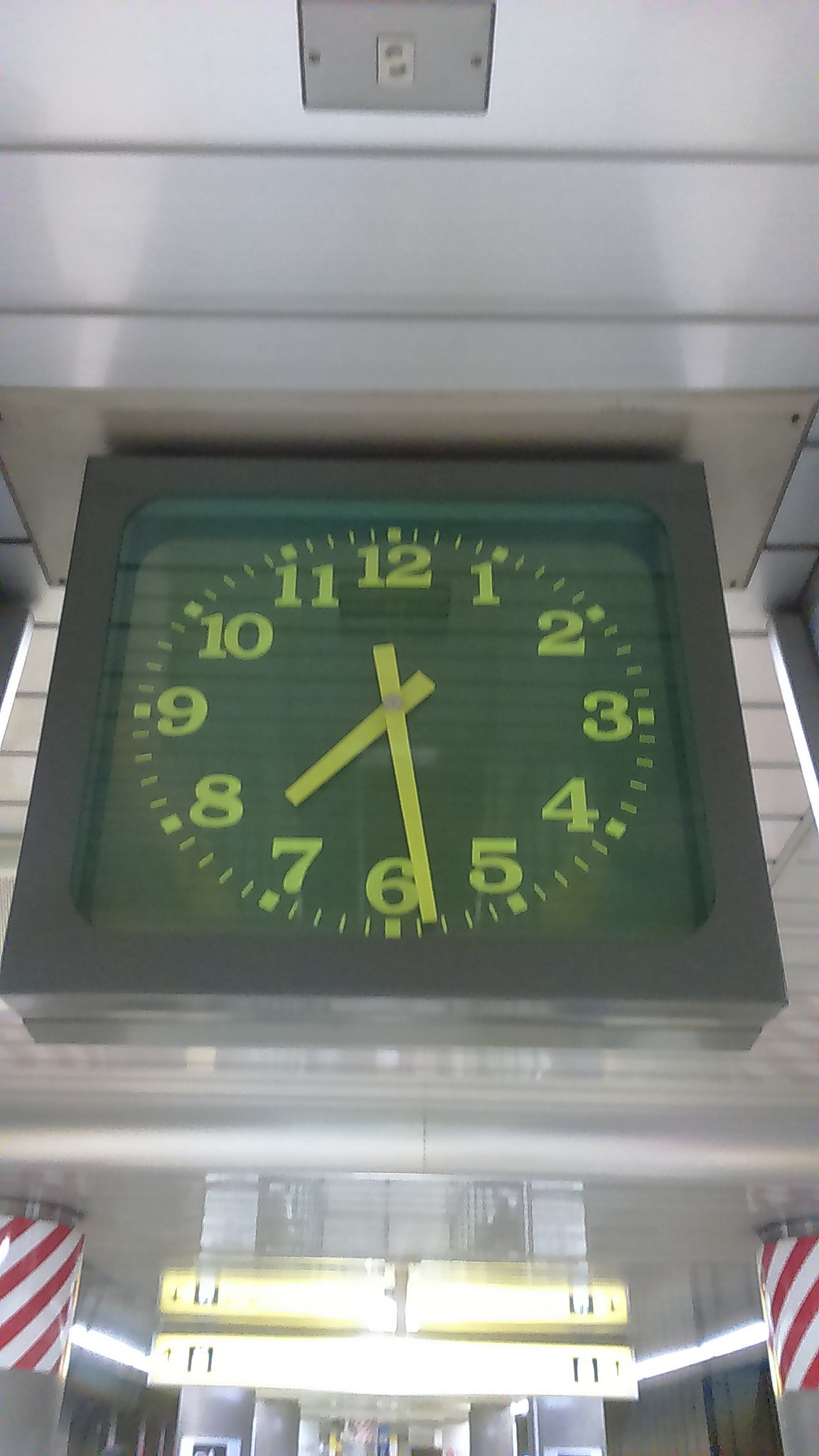The image, a narrow color photograph likely taken with a smartphone, prominently features a large analog clock mounted on a wall, occupying the central portion of the frame. The clock has a distinctive, dark brown square casing with a neon green dial. The numbers, also neon green, indicate the time at approximately 7:29, with the minute hand just one and a half increments before the six and the hour hand between the seven and eight.

The environment resembles a bustling, possibly underground train station or shopping area, characterized by numerous concrete pillars beneath the clock and a multi-level ceiling. Above the clock, the ceiling extends backward before dropping down, suggesting a higher level behind the camera. This spatial arrangement is typical of walkways found in underground stations. Illuminated signs, appearing as overexposed yellow rectangles, emphasize wayfinding, although their details are obscured due to the lighting.

Flanking the bottom left and right corners of the image are red and white striped poles, reminiscent of barber shop décor. The absence of people, writing, or animals in the image focuses the viewer's attention on the architectural elements and the striking neon clock at its center.